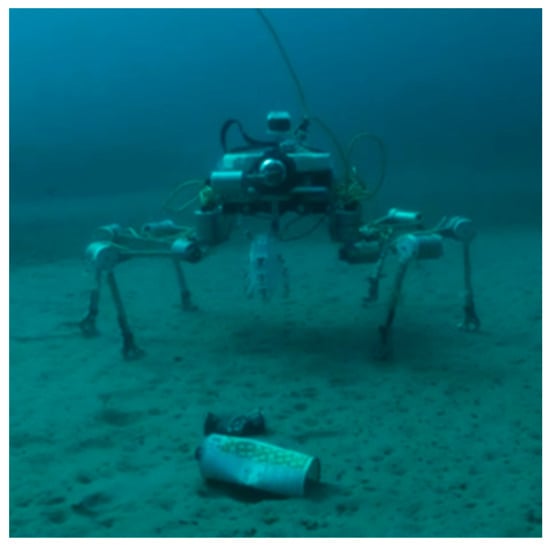The image portrays a remotely operated underwater robot resembling a metal spider with six articulated legs, each with two joints. It stands on a plain, sandy seabed devoid of coral or fish, moving towards a crushed aluminum can and another dark-colored piece of litter. The entire scene is bathed in a blue-green turquoise hue, creating a murky underwater atmosphere. The center of the robot hosts a network of coiled wires or cables, with one extending upward out of the frame. The robot, controlled from above the surface, features a clamp-like appendage capable of picking up objects. Shallow depressions in the sand likely mark the machine’s movements.